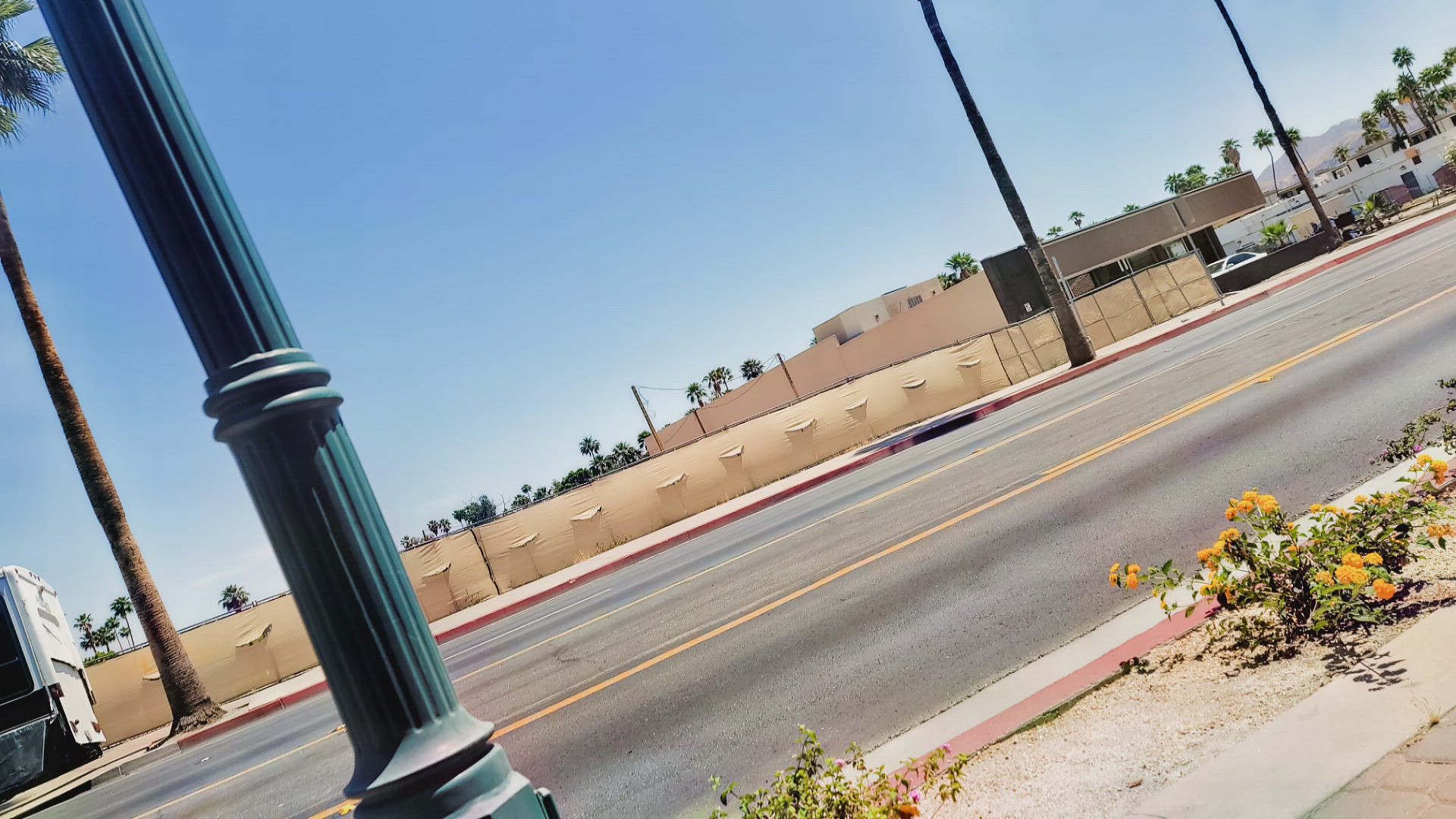This photograph captures a tranquil street scene devoid of moving vehicles, with only the rear end of a bus peeking into the lower left corner. The street is oriented diagonally across the frame, stretching from the lower left corner to the upper right. The foreground features a sidewalk bordered by a thin strip of dirt, hosting low-growing greenery and clusters of small yellow flowers. The road itself, marked by worn gray pavement and a central yellow dividing line, contrasts with the vibrant flora. A red curb runs along the far side of the road, adjacent to another gray sidewalk from which three tall palm trees ascend. The trunks of two palm trees dominate the right side, while the leftmost reveals a few fronds in the upper left corner. 

A dark green streetlight or signpost stands prominently in the foreground, aligning with the leftmost palm tree across the street. Behind the sidewalk on the opposite side, a beige-colored fence, likely a chain-link design covered with canvas or tarp, encloses the area. In the distance, more palm trees are visible, along with a low tan and brown building situated on the right. The sky overhead is a clear, soft blue, subtly fading to a lighter shade near the horizon, enhancing the serene ambiance of the scene.